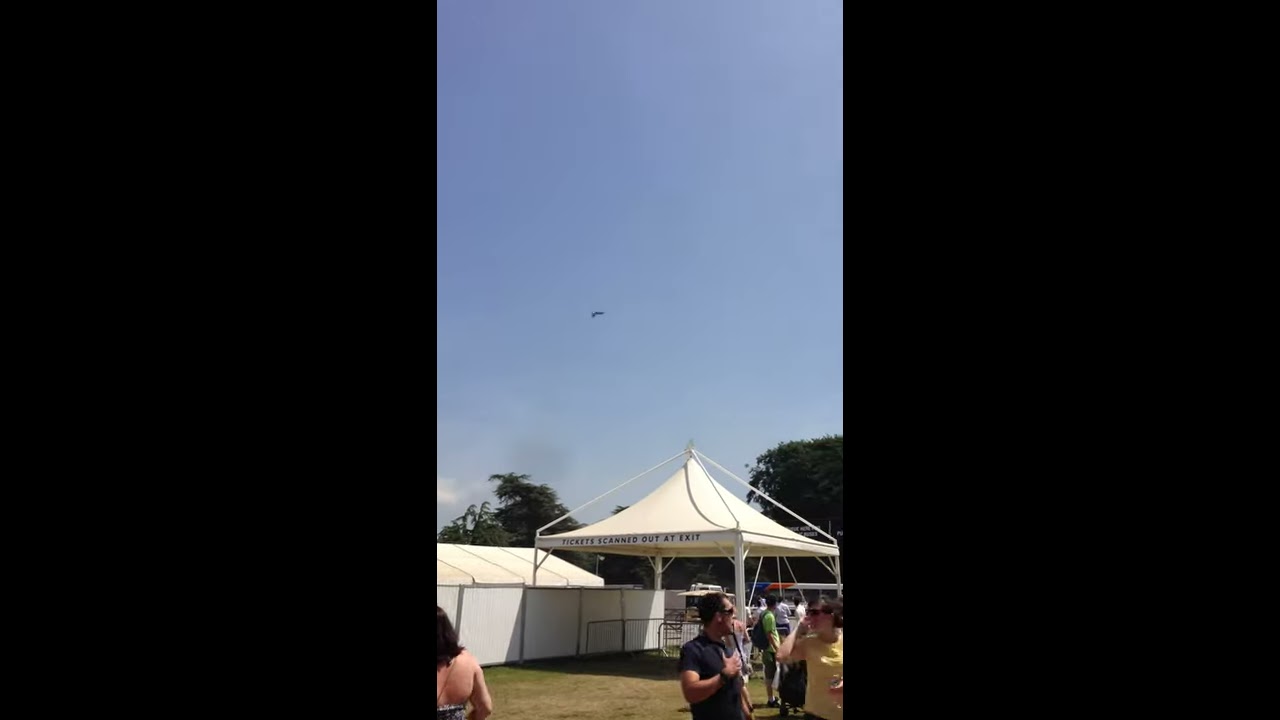The image depicts an outdoor festival setting, with groups of people standing and interacting in the lower third of the frame. A distinctive large white pop-up canopy tent is centered in the background, featuring bold black all-capital text that reads, "TICKETS SCANNED OUT AT EXIT." To the left of the canopy, you can see parts of a white building and some trees, while on the right, a mixture of buses, dividers, and other vehicles or equipment are visible. The ground is a mix of grass and dirt. Prominent in the lower left corner is a woman with shoulder-length dark brown hair, her back turned to the viewer, while on the lower right, a man in a black t-shirt and a woman in a yellow t-shirt can be seen. Above the tent and dominating much of the image is a clear blue sky, in which a lone drone is hovering approximately 10 to 15 feet above the canopy. The bright, sunny weather accentuates the festive atmosphere, with a hint of a plane or similar object faintly discernible in the distant sky.